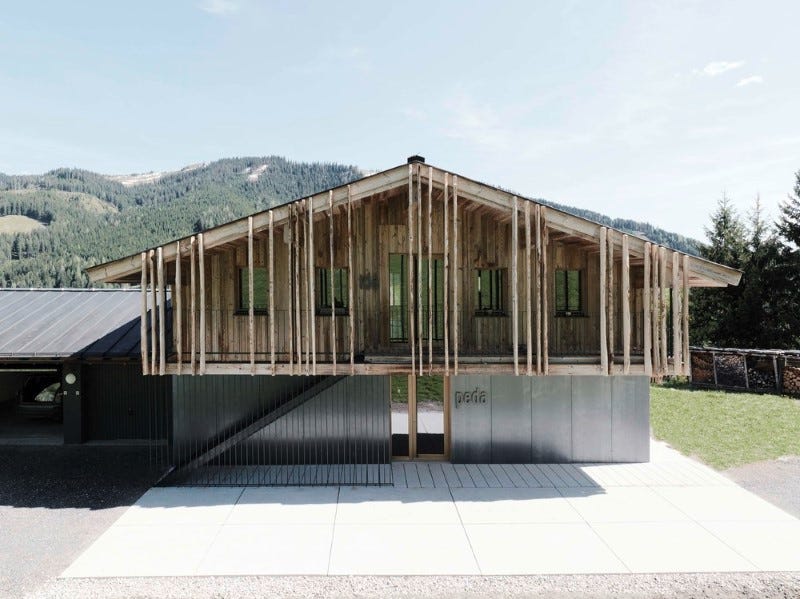This detailed outdoor daytime photograph captures a partially constructed two-story house, resembling an alpine chalet, centered within a mountainous landscape. The rectangular image, about six inches wide and four inches high, features the house elevated on a large concrete pad. The lower story is enveloped with metal framing and panels, including an open, shaded garage door to the left. The right-side bottom story includes visible wooden beams in an unfinished door area, with the word "PEDA" marked on one of the metal frameworks.

A stairway on the left side of the ground floor ascends to the second story, which prominently displays reclaimed wood forming its facade. The upper porch area is equipped with horizontal wooden beams and a metal fence railing. Visible inside, through the openings, are glimpses of furniture, potentially beds or dressers. In front of the structure lies a cement patio area with large white squares forming a driveway-like space. 

Surrounding the construction site are tree-covered hills in the background, providing a natural alpine backdrop. The scene is topped with a light blue sky, enhancing the tranquil yet industrious atmosphere.